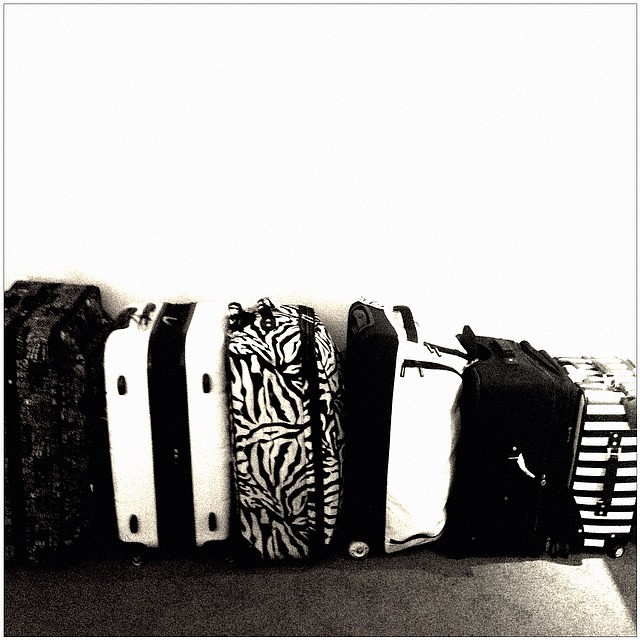The black-and-white image showcases a series of six suitcases lined up against a stark white wall with a black, carpeted floor that gradually fades to gray from left to right. Each suitcase varies in size and design, standing upright with visible wheels and handles for rolling. Starting from the left, the tallest suitcase features a black and white pattern that is somewhat indiscernible. Next is a hard case, predominantly white with a black middle section. Following that is a suitcase with a zebra-like stripe pattern or leaves. To its right, there's a bag split evenly into black and white halves, complete with black zippers. The fifth suitcase is completely black, short, and squat with a pull-up handle. The final suitcase on the far right is adorned with black and white pinstripes and has a small handle for carrying.